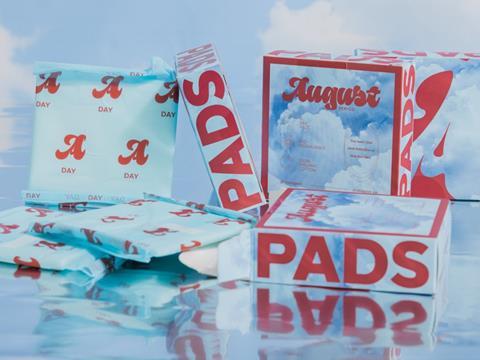The image displays four identically packaged boxes of August A-Day Pads, set against a backdrop of a clear blue sky with white clouds. Each square-shaped box features a white and red border, with the brand name "August" prominently printed in elegant red cursive on the front and the word "Pads" in bold, capitalized letters on all sides. The packaging also reveals individual blue, square-shaped bags, three of which are visible in the image, each marked with a large red letter "A" and the word "Day" below it in capital letters. The sky background is reflected on the surface where the pads are positioned, enhancing the serene aesthetic of the photograph.